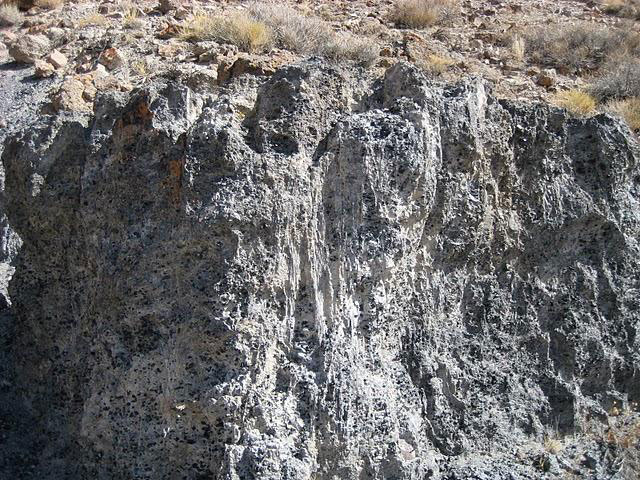The image captures a rugged, gray-colored cave or canyon wall characterized by its spongy appearance due to numerous air pocket-like holes. The stone wall exhibits a streaky pattern with a mix of white, dark gray, and light gray hues. At the upper part of the image, there is an assortment of dried grasses and small bushes in shades of brown, green, light gray, and light yellow, emphasizing the arid, desert-like environment. Sunlight hits the stone from the right, casting shadows on the left side, and highlighting its varied texture. The scene includes scattered debris around the vegetation, possibly small rocks or undetermined litter, contributing to the untamed feel of the terrain. The background suggests a significant drop-off behind a jagged ledge, hinting at the precarious nature of the landscape.